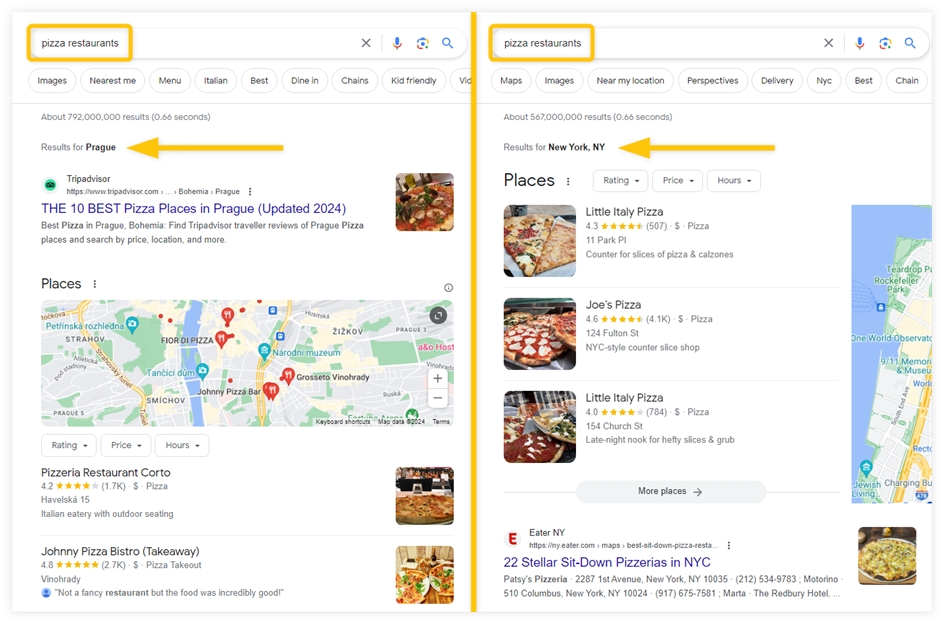The image displays a detailed side-by-side comparison of search engine results for "pizza restaurants," with a gold outline highlighting the words "pizza restaurants" in the search bar at the top of both pages. A gold line vertically divides the two webpages. On the upper sections of both pages, standard search engine features are visible: a close button (X), a blue microphone icon for voice search, a multicolored camera for image search, and the ubiquitous magnifying glass icon for initiating the search.

Directly below the search bar, the left page offers navigation options such as "images," "nearest me," "menu," "Italian," "best," "dine-in," "chains," and "kid-friendly." The right page presents slightly different options: "maps," "images," "nearby location," "perspectives," "delivery," "New York City," and "best chain."

The search results on the left side reveal approximately 792 million results returned in 0.66 seconds. The primary results highlight a suggestion to research pizza places in Prague, with "Prague" bolded and a yellow arrow pointing at it. On the right side, search results suggest pizza places in New York City, with "New York, New York" bolded and similarly accompanied by a yellow arrow.

In the left pane, top results start with a TripAdvisor link prominently labeled "The 10 Best Pizza Places in Prague (Updated 2024)," accompanied by TripAdvisor's green icon, a thumbnail image, and a listing of a few top pizza places. One such listing is "Pizzeria Restaurant Corto," rated 4.2 stars from 1.7k reviews, described as an Italian eatery with outdoor seating. Another entry is "Johnny Pizza Bistro (Takeaway)," boasting a 4.8-star rating from 2.7k reviews, and includes a user comment mentioning the food's quality despite the venue's simplicity.

The right pane showcases similarly formatted results for New York City. The first result is "Little Italy Pizza," rated 4.3 stars from 507 reviews, located at 11 Park Place, described as offering counter service for pizza slices. "Joe's Pizza," with a 4.6-star rating from 4.1k reviews, is noted for its New York City style pizza available at 124 Full Hand Street. Another listing for "Little Italy Pizza" at 154 Church Street has a 4.0-star rating from 784 reviews, famous for its hefty, late-night pizza slices.

Both pages also contain maps, which display local topographical elements like bodies of water, green spaces, and yellow pathways. Each map section appears just below their respective search results, offering visual cues for the location of the pizza places.

The right page further lists a specialized link from "Eater New York," suggesting "22 Stellar Sit-Down Pizzerias in New York," with detailed addresses, phone numbers, and a mention of locations such as "Patty's Pizza" and "Marta at the Redbird Hotel."

This detailed depiction encapsulates the nuances in search results, user interface elements, and differing context-rich results based on geographical focus between Prague and New York City, providing a comprehensive understanding of the search engine comparison presented in the image.